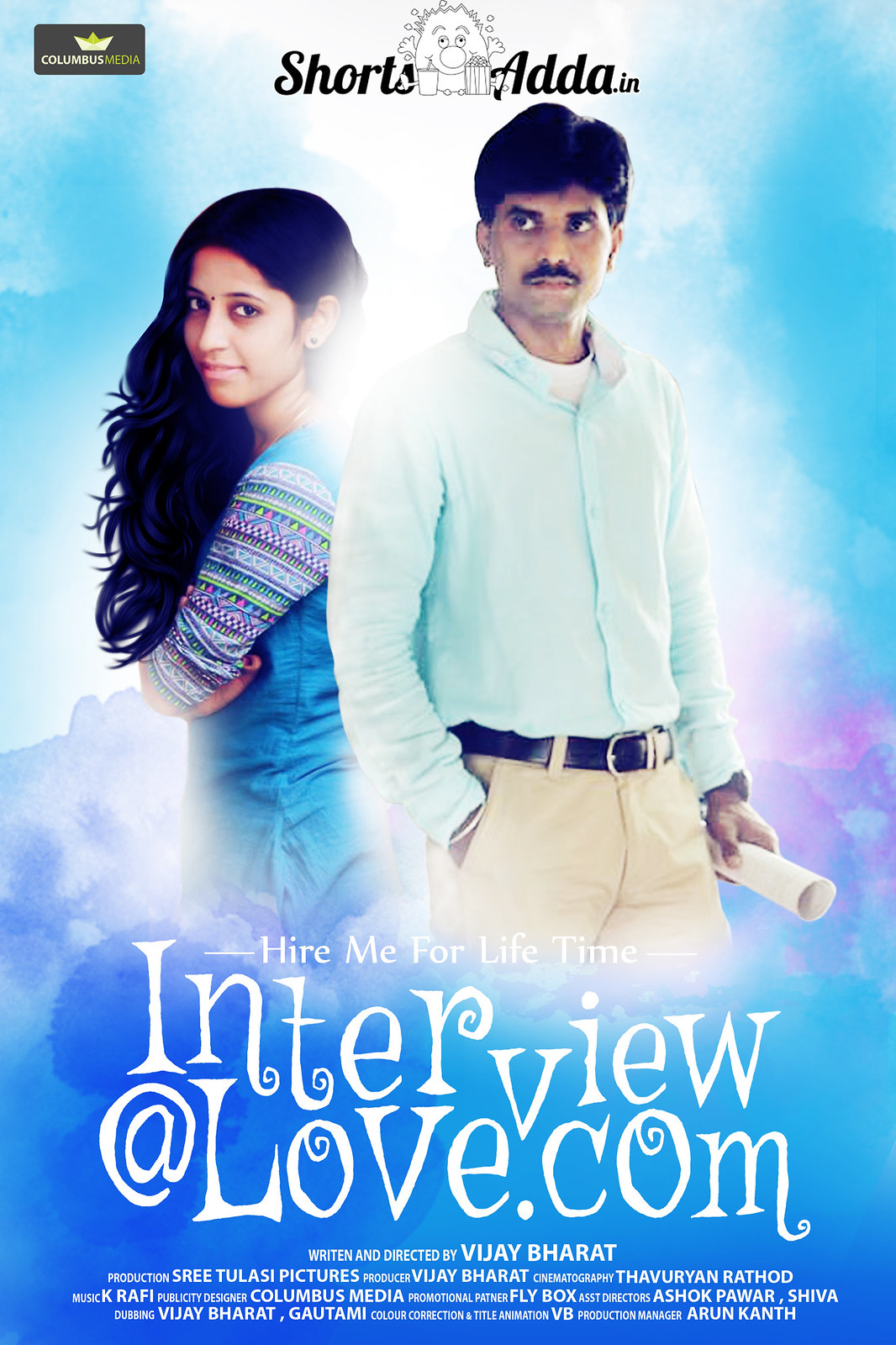The image is a promotional poster for an Indian movie titled "Hire Me for Lifetime," advertised on the Indian website Shortsadda.IN. In the upper left corner, the name "Columbus Media" is displayed alongside a green and white crown logo. The focal point of the poster features an Indian couple standing back-to-back. The man, wearing a blue collared shirt and brown pants, holds a rolled-up piece of paper and has mid-length black hair with a mustache. The woman, who has long dark brown hair, wears a turquoise and purple shirt with a striped design, and denim. The background of the poster consists of a blue sky with clouds, giving it a heavenly look. Below the main image, the text "Hire Me for Lifetime" appears in white, followed by "interview at love.com" written in a fancy script. Additionally, the poster details the film's creators, including the writer and director Vijay Bharat, and other production credits such as cinematography, music, and title animation.